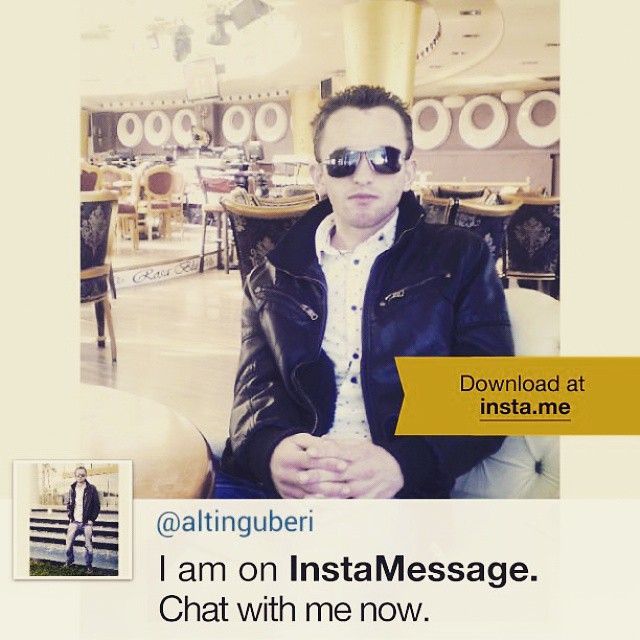The image depicts a young Caucasian man, possibly an entertainer, seated in an upscale restaurant or cafe. He has short, spiky brown hair with a pronounced cowlick in the center, and he's wearing mirrored sunglasses, a black leather jacket, and a white shirt. Sitting in a white chair, his hands are calmly intertwined on his lap, giving off a relaxed demeanor. In the background, there are additional chairs and tables, suggesting a busy setting like a mall or dining area. 

Overlaying the bottom right of the image is a yellow banner that reads, "Download at insta.me." Below the main photo, a smaller image shows the same man standing in front of a fence or steps under a sunny sky, wearing the same outfit and glasses. Beside this smaller picture, the text reads, "@ALTINGUBERI. I am on Instamessage. Chat with me now."